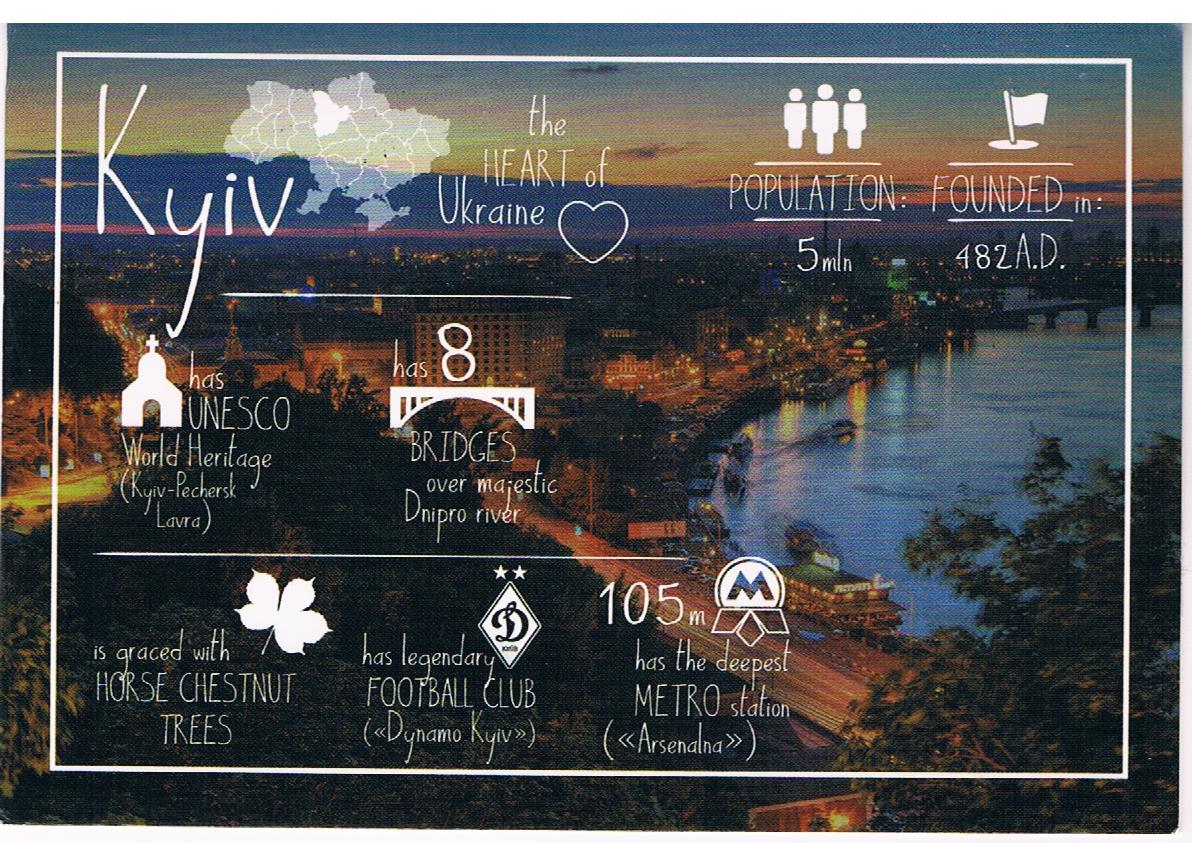The image is a detailed graphic, seemingly designed in PowerPoint, that presents a postcard-like view of the city of Kiev during the evening. To the right, a serene body of water, possibly part of the Dnipro River, stretches under the twilight, with the skyline of Kiev illuminated by city lights creating a warm, golden glow. In the distance, you can spot the city's diverse infrastructure, highways, and patches of woodland. The scene is overlaid with a variety of white handwritten fonts and illustrations. Prominently, it features key information such as "Kiev - The Heart of Ukraine" alongside a small heart icon, and highlights on a map showing Kiev's location within Ukraine. Additional details include the city's population of 5 million, its founding year of 482 AD, and notable features like the presence of horse chestnut trees and the legendary Dynamo Kiev football club. Icons and annotations further mention the UNESCO World Heritage sites and the eight bridges spanning the Dnipro River. The graphic combines a picturesque visual with informative text, making it both a beautiful and educational depiction of Kiev.